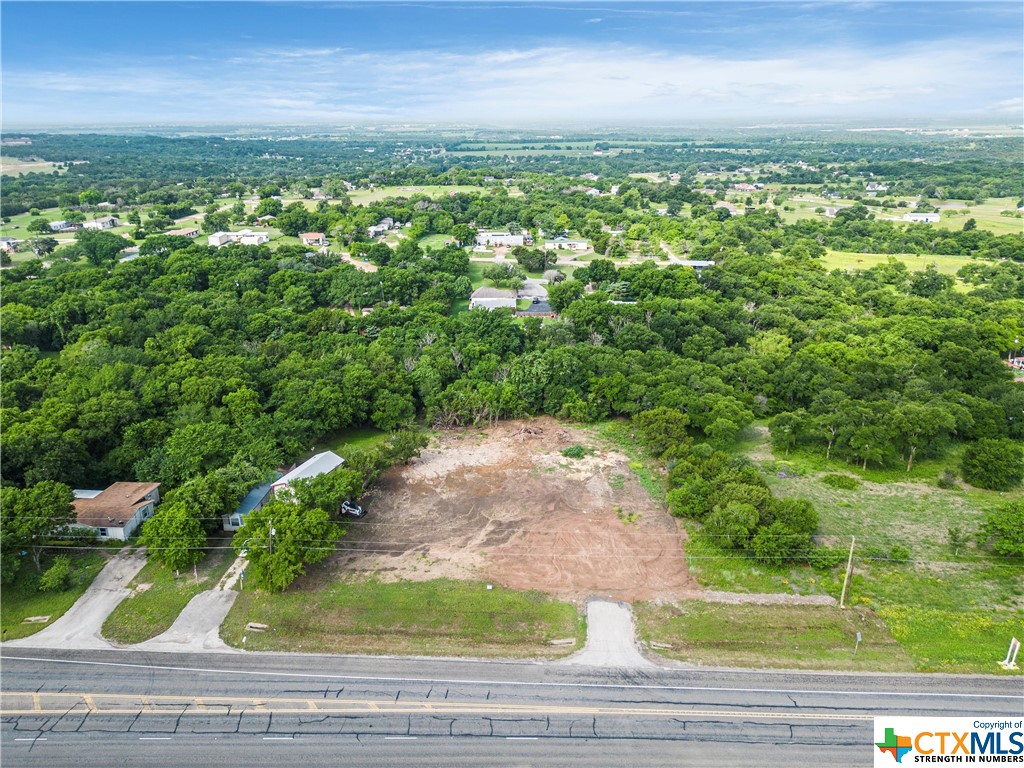This realistic, bird's-eye aerial view, likely captured from a drone, helicopter, or tall tower, showcases an expansive landscape stretching for miles. In the foreground, a cracked macadam road runs diagonally across the bottom of the image, lined with three driveways. The left driveway leads to a small house with a brown roof, while the middle driveway reaches a longer gray house with a blue roof. The rightmost driveway extends into an empty, cleared lot with a small tractor, indicating future construction.

Surrounding these driveways, the landscape is predominantly forested, with dense tree canopies masking the ground below. In the middle distance, another road runs horizontally across the image, flanked by additional houses and buildings, interspersed with more trees. This pattern of clustered buildings amid vast greenery extends into the horizon, where scattered neighborhoods and further stretches of forest can be seen under a bright, sunny sky partially covered by clouds.

At the bottom right corner of the image, there is a small white rectangle featuring the text "copyright of CTXMLS, Strength in Numbers," accompanied by a graphic of Texas divided into four colored regions by black lines.